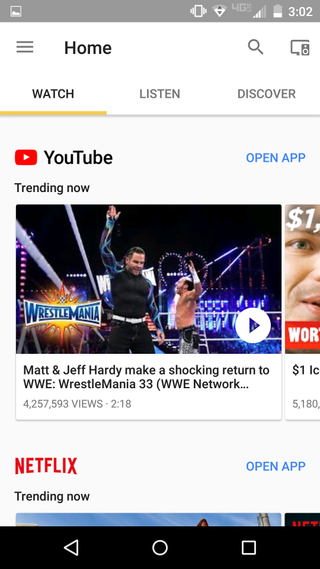This image depicts a website interface being viewed on a smartphone that promotes both YouTube and Netflix content. The top of the page features a "Home" label along with a search bar. The screen displays the option to "Watch, Listen, Discover." The first section is dedicated to YouTube, with the " YouTube " label prominently written in black. Below this, a blue button prompts users to "Open App," and the section titled "Trending Now" reveals current popular content. Featured is an image of WWE wrestlers Matt and Jeff Hardy, noting their "shocking return to WWE" at WrestleMania.

Directly beneath the YouTube section is the Netflix segment, marked by the iconic red Netflix logo. Here, users also have the opportunity to "Open App" via a blue button. Another "Trending Now" section follows, displayed in black text. Although partially obscured, the visible portion includes a blue sky with some indistinct objects. The bottom of the phone screen shows various app icons, completing the intuitive and streamlined display.